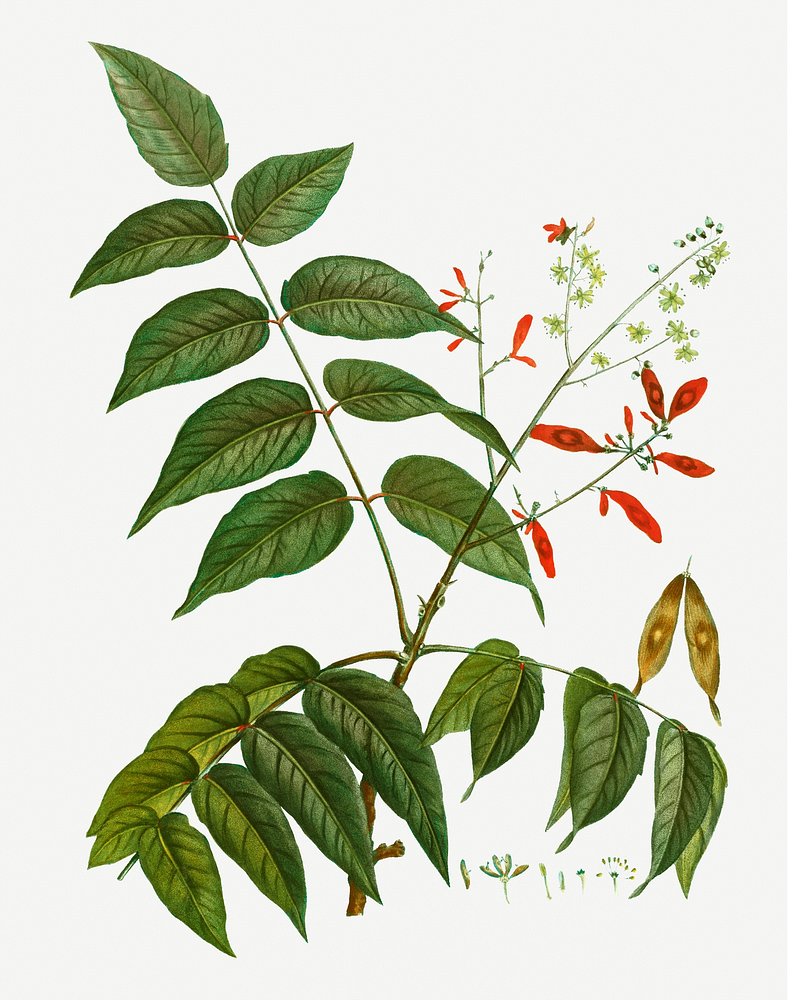This detailed colored pencil drawing depicts a tree branch on a white background, showcasing various stages of its life cycle. The composition features a central stem from which several smaller branches spring. Dominating the lower and middle parts of the stem are clusters of large, dark green leaves. 

As the eye travels up the stem, a significant branch extends to the right, adorned with striking red flowers. Above this, more red flowers intermingle with tiny green flowers, demonstrating a progression towards the mature foliage at the top of the drawing. In the upper section, near the extremities, the branch showcases small green, star-shaped leaves and mint-green buds, representing the new growth of the plant.

The lower corners of the picture feature additional details: the bottom left corner has lighter green leaves that mirror the ones above, while the bottom right corner displays some little buds beneath another leafy stem. This intricate illustration not only captures the essence of a tree branch but also hints at the plant's growth stages, from budding to full bloom.